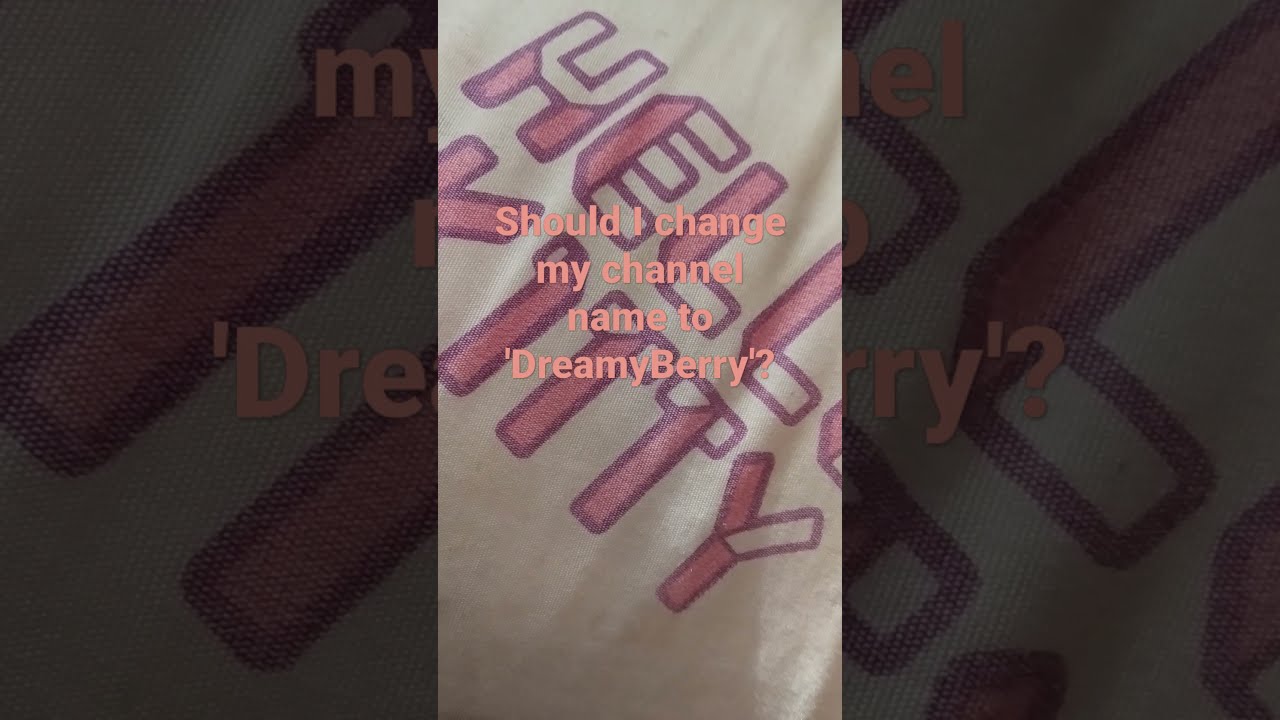In the image, there is a white cloth, likely part of a shirt, prominently featuring the iconic phrase "Hello Kitty" in large, pink and white block letters. However, some portions of the letters are cut off: the 'O' in "Hello" and the 'K' in "Kitty" are partially obscured. The 'H' in "Hello" is distinguished by having white at the top and pink at the bottom, while the 'E' has pink on the left side with its horizontal lines in white. The 'Ls' in “Hello” have pink vertical lines and white horizontal lines, and the word “Kitty” is mostly in pink with the tops of the 'Ts' in white. The image is divided such that the main focal point occupies the central third, with the left and right thirds showing parts of this central focal area.

Overlaying the "Hello Kitty" text, there is peach-colored text asking, "Should I change my channel name to 'Dreamberry'?" The word 'Dreamberry' is emphasized with single quotes and a question mark at the end. The background of the entire image is a light tan color and features a noticeable fold, further suggesting the material pictured is fabric, likely a shirt. The overall design gives an impression of the Hello Kitty brand combined with a personal query about rebranding.